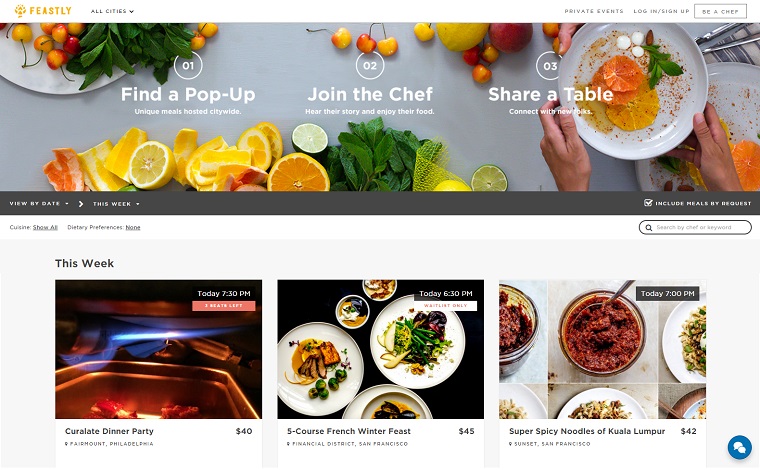Here is a refined and highly detailed caption for the image:

---

This is a screenshot of the Feastly website, displayed horizontally in the upper left-hand corner of the screen. The Feastly logo, highlighted in yellow, is prominently placed on the left side of the navigation bar. Next to it, "All Cities" is listed. On the far right of the navigation bar, there are options for "Private Events," “Log In,” and “Sign Up,” with a small rectangle indicating "Be a Chef."

The top of the page features a photographic banner with a gray background, displaying an enticing array of food, fruits, and vegetables. On the right side of the banner, coming from the lower right-hand corner, two hands are holding a round white plate topped with orange slices, mint leaves, and an orange sprinkle garnish. The bottom of the banner showcases a vibrant assortment of fruit slices, including oranges, grapefruits, and limes, complemented by additional green mint leaves. In the top left corner of the banner, a white plate holds yellow and red cherries alongside more mint leaves. 

Centered on the photographic banner is the text, "Find a Pop-Up, Unique Meals Posted Citywide. Join the chef, hear their story, and enjoy their food. Share a table, connect with new friends" (some text is partially obscured).

Below the banner, navigational options read "View by State," "This Week," and "Include Meals by Request." 

At the bottom of the page, three square images are displayed. The left image is titled "Curilate Dinner Party." The center image, "Five-Course French Winter Feast for $45," depicts three plates of elegantly presented food. The right image, "Super Spicy Noodles of Koala Lumpur," features a vibrant collage of six photos arranged in two rows of three, each displaying colorful and appetizing dishes.